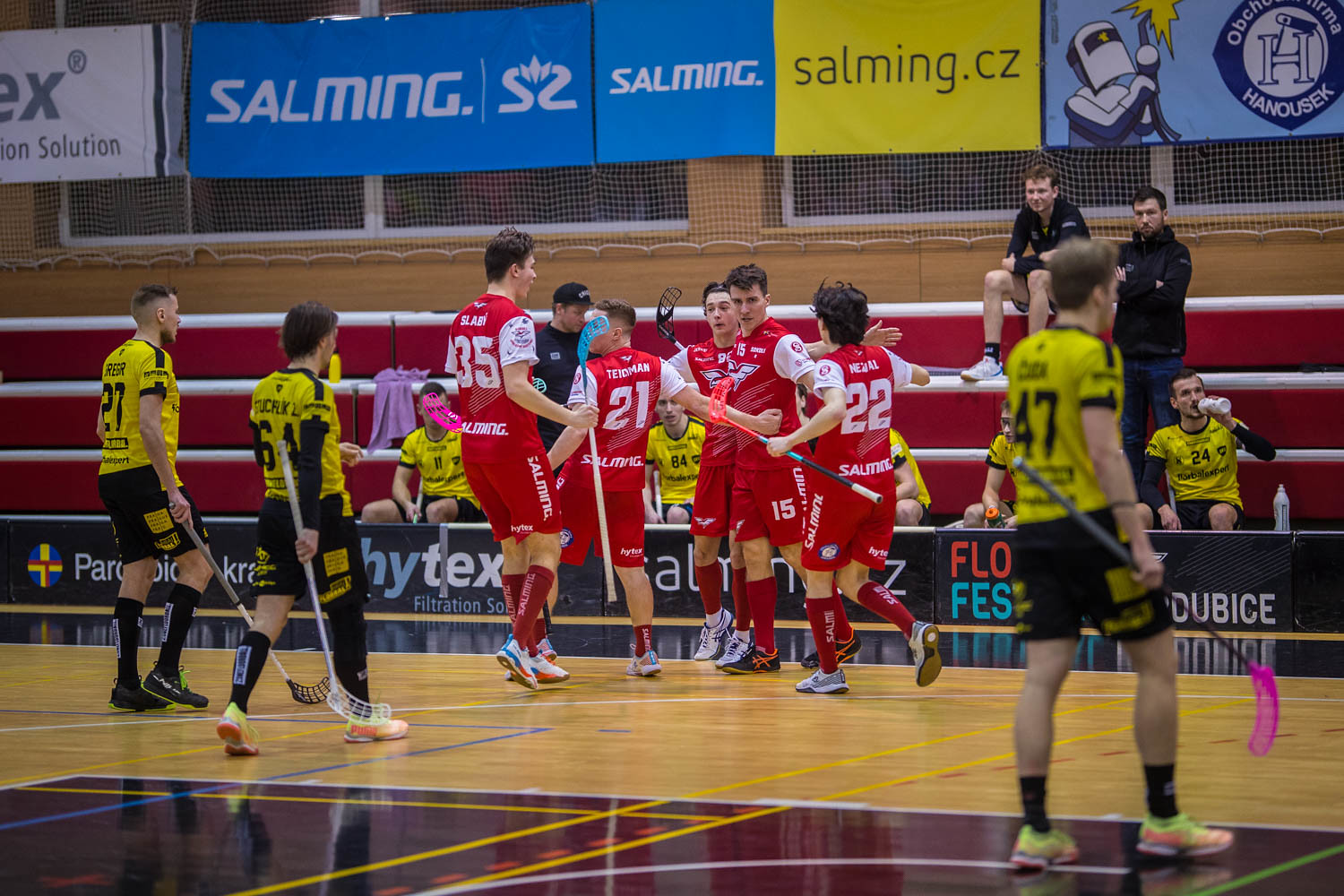This indoor sports arena features a polished wooden floor with visible paint markings. At the center, a group of athletes dressed in variously colored jerseys are engaged in what appears to be a lacrosse game, each wielding a lacrosse stick. Spectators can be seen seated on benches along the far wall, which is adorned with windows and several sponsor banners, albeit in an unreadable foreign language. The vibrant color palette includes maroon, white, gray, yellow, orange, blue, black, pink, and purple, adding to the lively atmosphere of the mid-day sporting event.